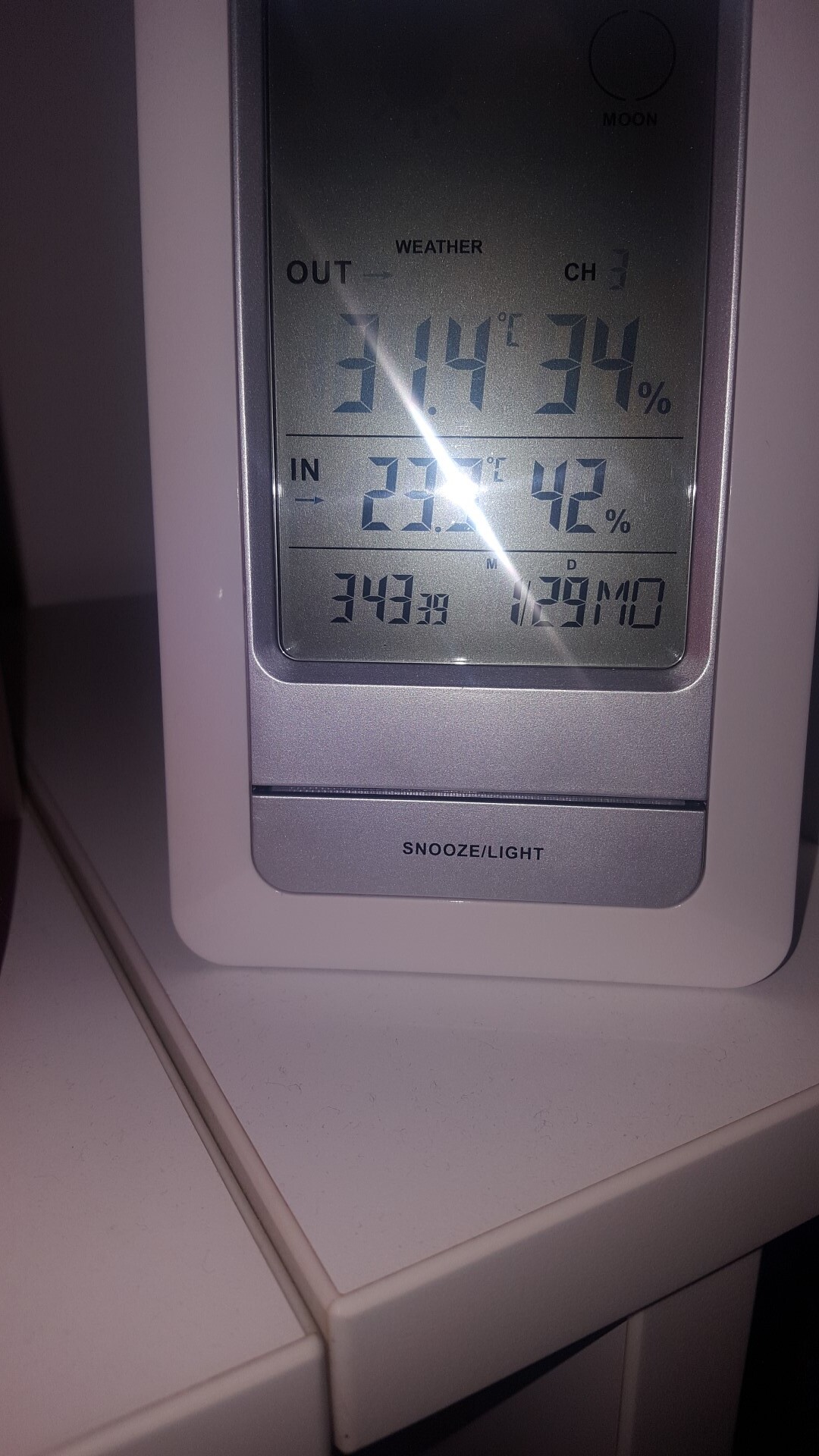In the foreground of the image, there's a digital electronic device displaying various readouts on its LCD screen. The top portion of the screen appears to be blank or inactive. The lower section features several readouts:

- A header bar labeled "WEATHER" in bold, uppercase black letters.
- Just below the header, it displays "CH 3," which likely indicates the channel number.
- A large bold number "31.4" followed by a degree symbol and a capital "C" denotes the current temperature in Celsius.
- The number "34%" follows, presumably representing the relative humidity.
- A horizontal line divides the sections, underneath which is the label "IN" in uppercase, followed by a right-facing arrow.
- Below that, the screen shows "32.3°C" reflecting another temperature reading.
- Another relative humidity readout shows "42%."
- Near the bottom, the display reads "C 343" followed by "39" in smaller numbers, possibly indicating barometric pressure or another metric, though it's not explicitly labeled.

To the right of these sections, another block displays:
- An "M" above "1" (likely denoting the month), followed by a forward slash and then "D" above "29" (indicating the day of the month).
- The display also shows "MO" which likely signifies Monday.

At the bottom of the device, it reads "SNOOZE LIGHT" in uppercase black letters, indicating buttons for a snooze function or backlight activation.

The LCD screen has a dark green-black background, bordered by a gray plastic frame. The device rests on a table with a white border that appears either unclean or textured with squiggly lines. The lighting in the room appears to be dim, likely sourced from the phone's camera, casting a glare on the LCD screen. To the left of the device, there's a white wall that appears dark due to the low lighting.